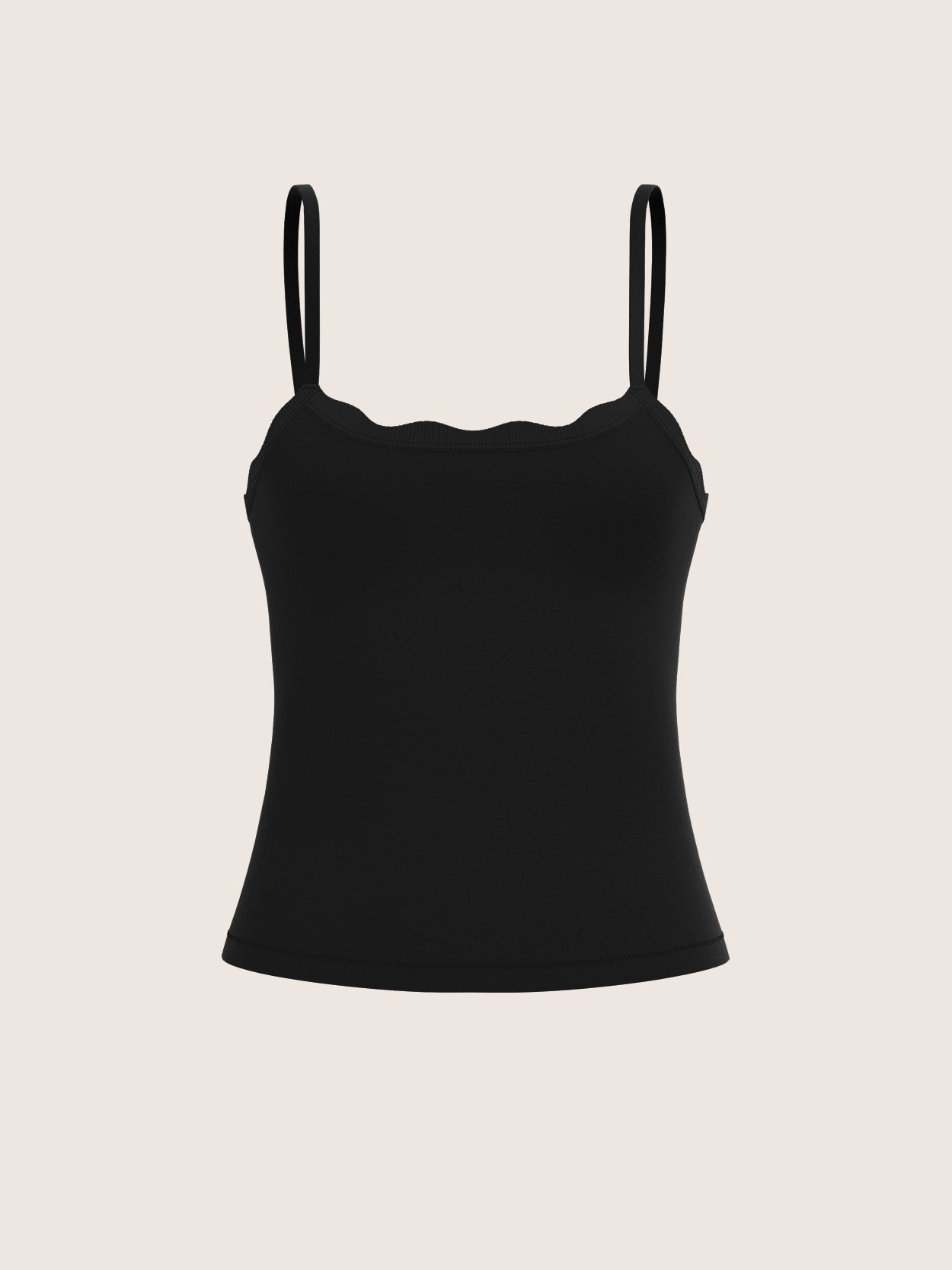This is a digital image of a woman's black camisole or tank top, showcased against a plain beige or tan background. The top features spaghetti straps that are fairly thin and looped, resembling bunny ears. It has a distinct wavy neckline rather than a conventional v-neck or scoop neck. The fabric appears to be stretchy, suggesting it would be suitable for activities such as yoga, ballet training, dancing, or other active pursuits. The shirt widens at the hips and tapers towards the bottom, with a wavy design below the neck area. It is a plain solid black color without any graphic designs or text, standing out sharply against the background, almost like a silhouette.